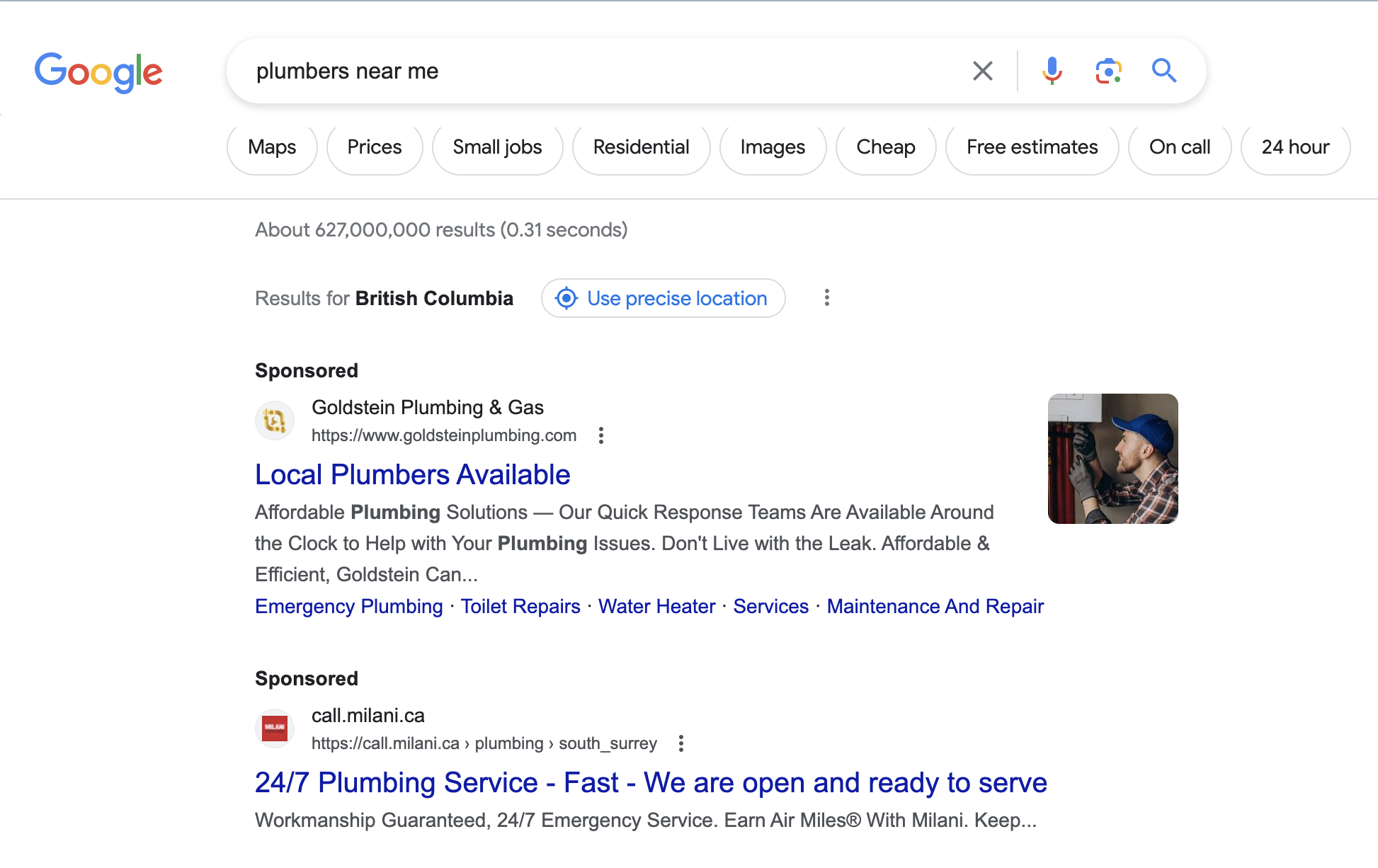The image depicts a Google web search page. On the left-hand side, the Google logo is prominently displayed in its iconic blue, red, yellow, and green letters. In the search bar, the query "plumbers near me" is entered. Next to the search bar are icons for a microphone, a camera, and a magnifying glass for initiating the search.

Below the search bar, there are various related search suggestions including "maps", "prices", "small jobs", "residential", "images", "cheap", "free estimates", "on-call", and "24-hour". The page then indicates that the results are specific to British Columbia, and there is a clickable option in blue text to "use precise location."

The first result is a sponsored ad for "Goldstein Plumbing and Gas," which advertises local and affordable plumbing services with quick response teams available around the clock. The ad urges potential customers not to live with leaks and highlights services such as emergency plumbing, toilet repairs, water heater services, and maintenance and repair. The ad includes a picture of a plumber wearing a baseball cap, a plaid shirt, gloves, and holding a tool.

The second sponsored result is for "CallMalani.ca," which also offers 24/7 plumbing services and assures fast, ready-to-serve assistance.